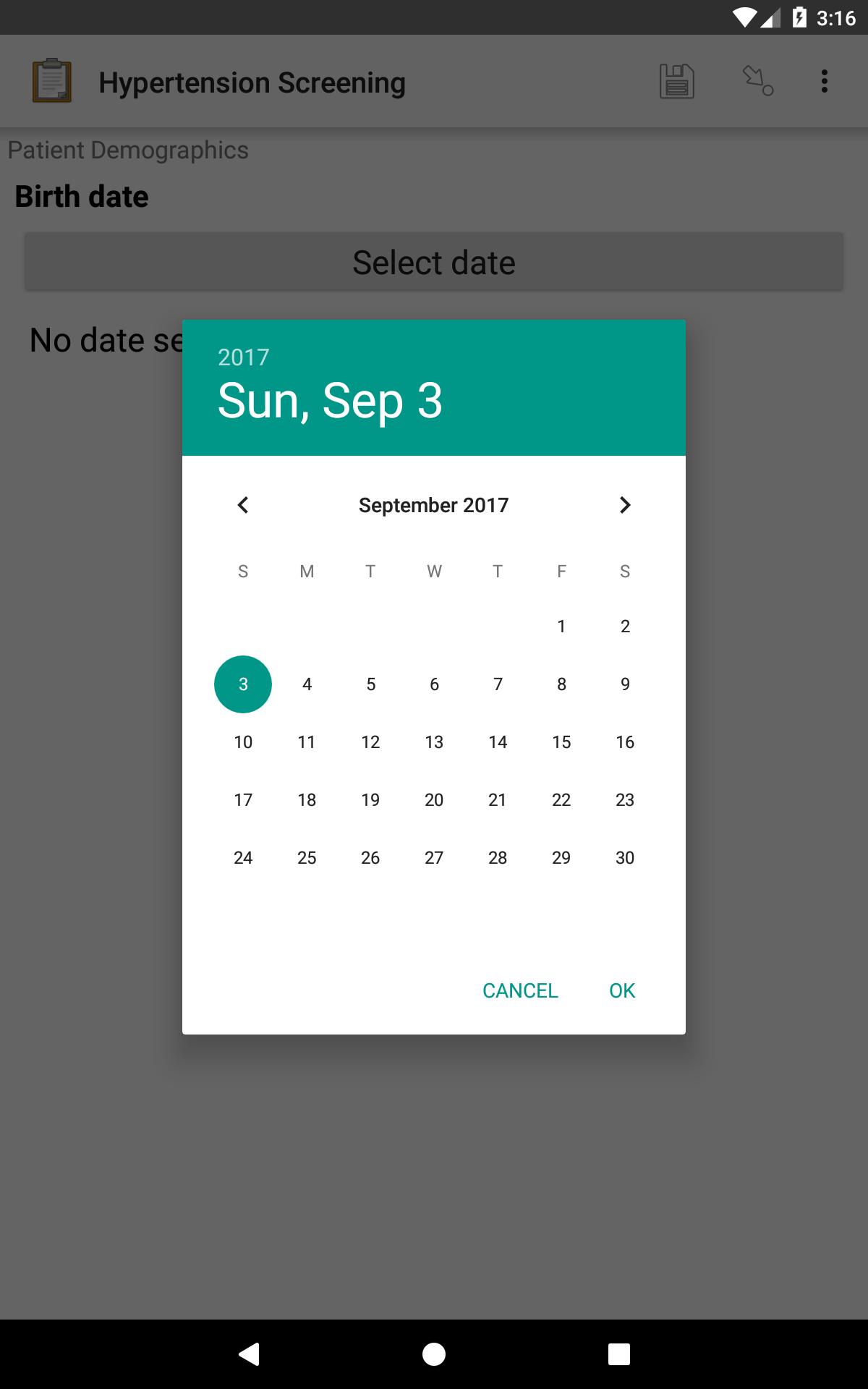The image depicts a smartphone screen displaying a website related to healthcare, specifically focusing on hypertension screening. The device is connected to WiFi, and the battery is fully charged, with the current time shown as 3:16. In the upper left corner of the screen, there is an icon resembling a clipboard, indicating that it pertains to medical records or notes. Next to this icon is another symbol, reminiscent of an old floppy disk, suggesting options to save or download information. An arrow and three dots are also visible, likely offering additional settings or more details.

Beneath these icons, the text "Patient Demographics" is displayed, followed by fields for entering patient information. Under the "Birth Date" field, there is an option to "Select Date," which triggers a calendar pop-up. This calendar features a teal-colored top border with the year "2017" prominently shown. The calendar is set to September 2017, with the specific date of Sunday, September 3rd, highlighted in green. The days of the week and corresponding dates are clearly lined up in the conventional calendar format for that month and year.